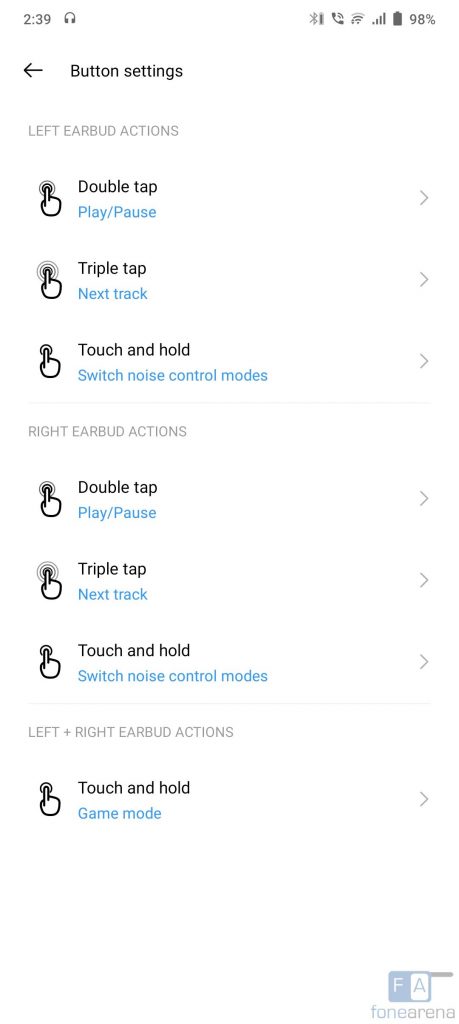This image displays a mobile user interface designed for managing earbud actions. At the top of the screen, the standard phone interface is visible, showing the time, reception bars, battery level, and internet connection status. Below that, the interface is labeled "Button Settings," with a left-pointing arrow for navigating back.

The main section is divided into three parts: "Left Earbud Actions," "Right Earbud Actions," and "Left & Right Earbud Actions." Each section allows users to customize various controls. For the individual left and right earbuds, users can program actions such as double-tap to play/pause, triple-tap to skip to the next track, and touch-and-hold to switch between noise control modes. The combined earbud actions section includes an option to touch-and-hold for activating game mode.